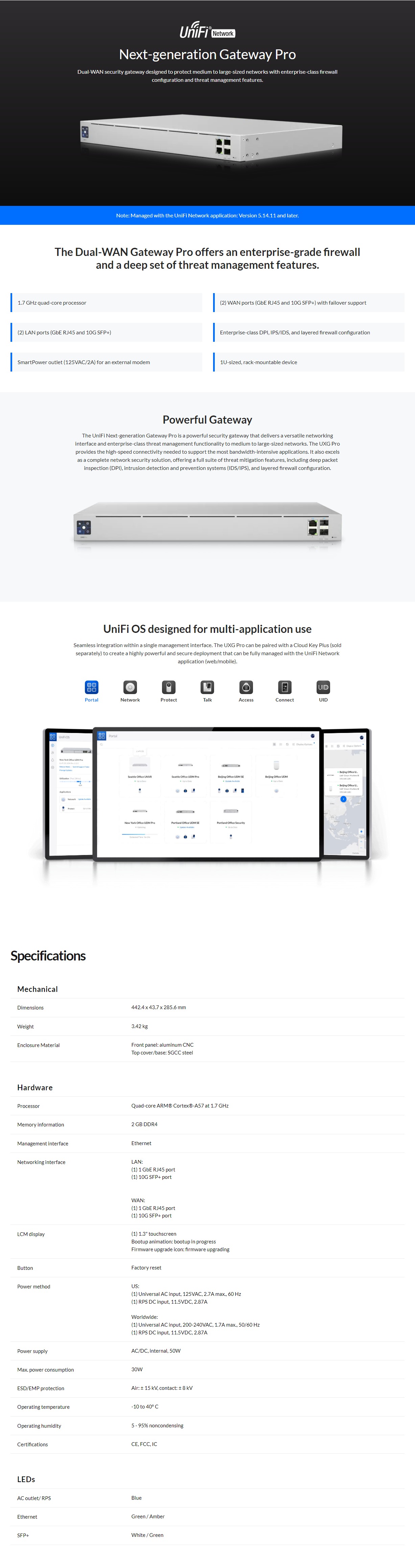This image showcases the Unifi website, distinctly spelled as "U-N-I-F-I." The website is displayed in a compact view, making the fine print challenging to read. At the top of the page, there's a black banner with a blue stripe at its bottom, featuring the text "Next-generation Gateway Pro." Below this banner, there is an image of a white box with a black right side, adorned with a logo on the left.

Accompanying the image, the text reads, "The Dual WAN Gateway Pro offers an enterprise-grade firewall and a comprehensive set of threat management features. This powerful gateway utilizes the Unified OS, designed for versatile application use." 

The page also displays various images set in tiles, icons, and descriptive text. Further down, there are screens showing the OS in action, seemingly on tablets. Near the bottom of the image is a section labeled "Specification," presenting a detailed list under categories titled "Mechanical" and "Hardware," with an additional category for "LEDs" near the bottom.